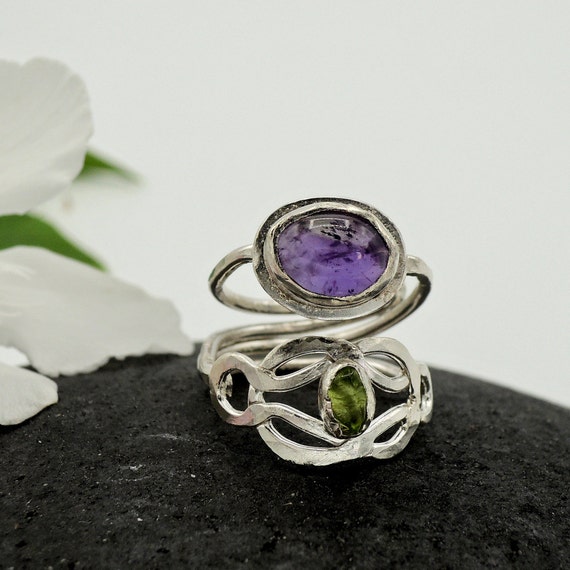This close-up image captures a beautifully intricate piece of jewelry comprised of two parts. The central piece features an S-shaped design, reminiscent of a coiled snake, and prominently showcases an oval-shaped amethyst stone at its core. This amethyst exhibits strikingly dark flecks that add to its allure. Attached to this is a secondary ring that tapers off into a light green emerald or similar stone, resembling the shape of a human eye. The entire piece is crafted from silver, with detailed swirling motifs along the base and a simpler frame for the amethyst gem. These pieces of jewelry are positioned on a dark, possibly black rock surface, enhancing the vivid colors of the stones. To the left of the jewelry, there is a white flower with green petals, which is artfully blurred to keep the focus on the rings.